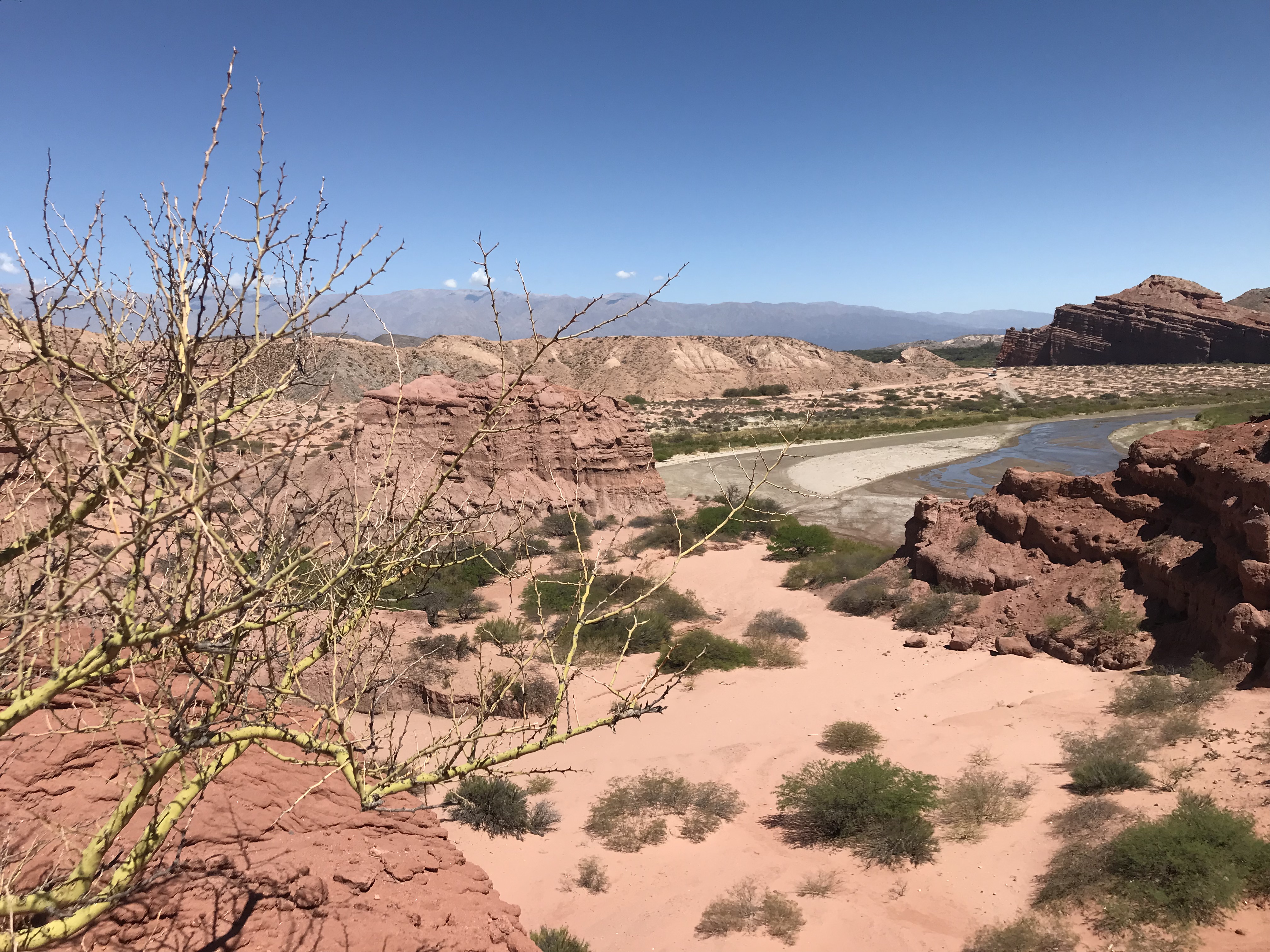This image depicts a vast, arid landscape resembling a desert. The ground is covered in sand of various brown hues, scattered with numerous rocky formations. Dominating the foreground is a tree without leaves, its branches stretching outward in a lifeless manner, tinged with yellowish and greenish shades likely due to sunlight reflection. Nearby, several small green shrubs dot the dry terrain, struggling to survive in this harsh environment. To the right of the image, there is a patch of water, suggesting a nearly dried-up river, hinting at the arid climate. The background features towering, rugged mountains against a clear, light blue sky, with a few clouds perched atop them, enhancing the desolate beauty of this desert-like scene.